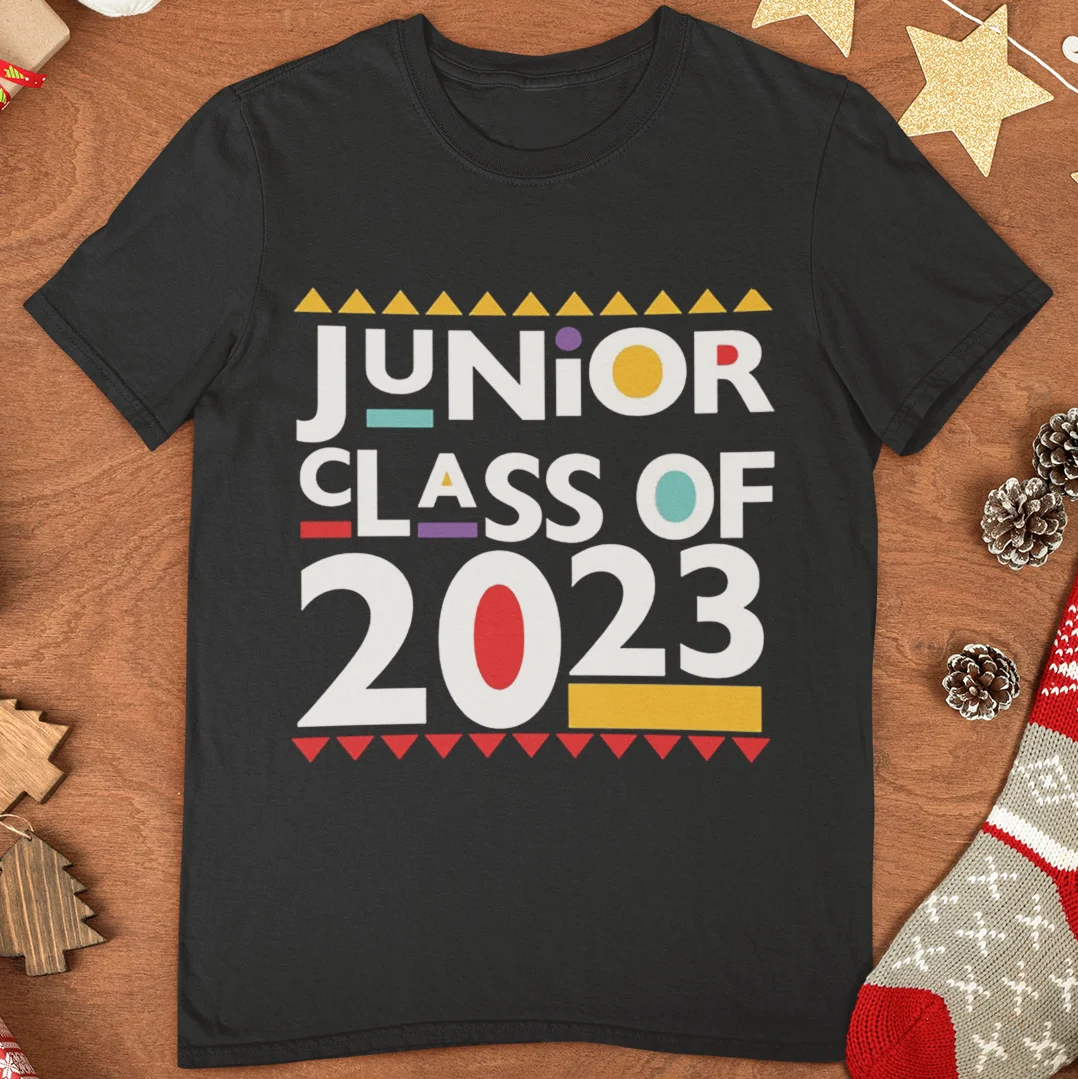The image depicts a nearly square photograph set against a wooden background adorned with festive items. Dominating the center is a black t-shirt that reads "Junior Class of 2023," with vibrant lettering in a mix of white and various colors. Yellow and red triangles adorn the top and bottom sections of the text, respectively. The individual letters and numbers are creatively accentuated: the '0' and 'O' are filled with red and yellow, the 'U' is underlined in blue, and additional shapes in turquoise blue, purple, red, and yellow underline other characters. Surrounding the shirt, the rustic wooden backdrop hosts several Christmas-themed decorations. On the right, there are three pinecones dusted with white, mimicking snow, and a red, gray, and white stocking in the corner. To the left, wooden ornaments and a piece of ribbon-tied wood are partially visible. The top right corner features paper stars strung together, adding a touch of holiday cheer to the scene.